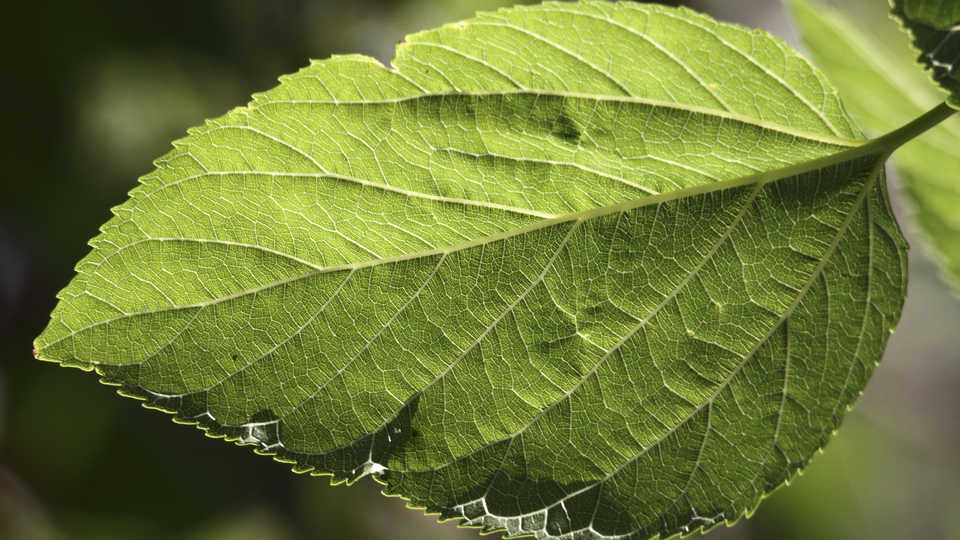This close-up photograph captures the intricate details of a single green leaf taken from its underside. The leaf is perfectly zoomed in, showcasing its intricate vein structure, with a central vein splitting the leaf in half and smaller veins branching outwards. The upper half, bathed in sunlight, is a lighter green, while the bottom half appears in a darker shade of green, almost black near the tip. The edges of the leaf have a slight watery residue, suggesting it has been wet. The background, though blurred to emphasize the leaf, reveals hints of other leaves and indistinct masses of black, grayish-white, and brown, adding depth and contrast to the image. Overall, the focus on the leaf's texture and the subtle play of light and shadow create a visually captivating scene.